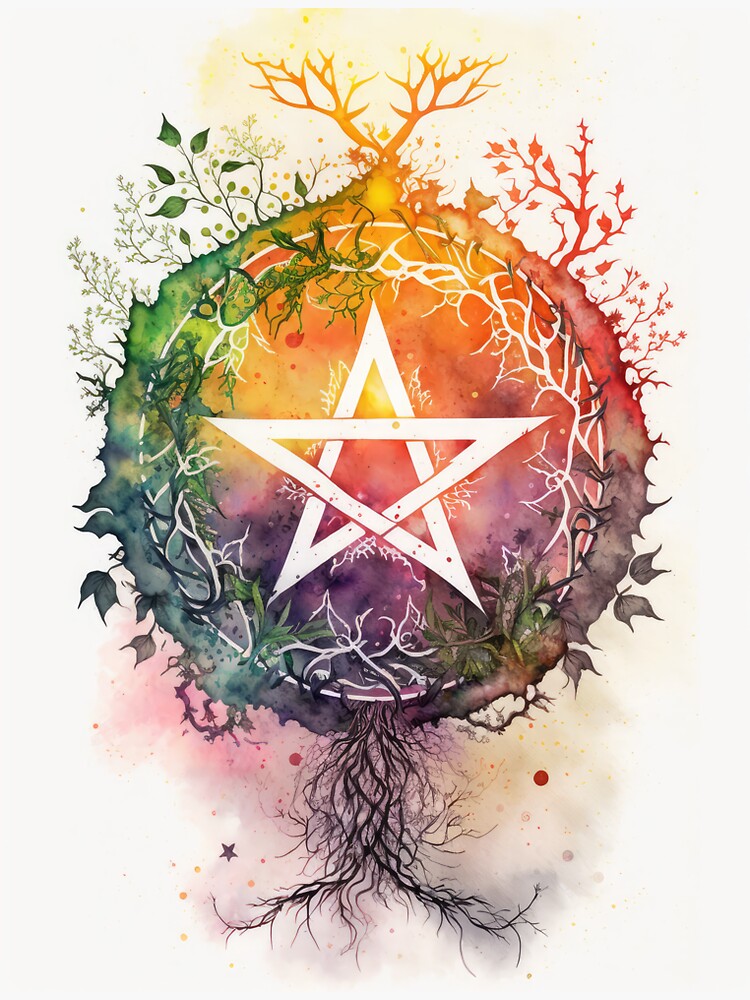The image is a portrait-oriented watercolor illustration, with a highly detailed and colorful design. At the center of the composition is a white pentagram, enclosed within a white ring. Surrounding this central element is a multi-colored circular background, featuring a gradient of greens and blues on the left, transitioning to reds, oranges, and yellows at the top, and purples and pinks towards the bottom right.

Encircling this vibrant backdrop is an arrangement of various trees and plants. On the left, there are green and blue trees, while the right side showcases red and purple foliage. At the top, an orange tree extends upward, complemented by a network of leaves that integrate into the design. The bottom part of the circle features an intricate root system drawn in black, blending into a light wash of pink, orange, and purple watercolor. Star shapes and circles accentuate the background, providing an ethereal touch.

Overall, the illustration is a harmonious blend of natural elements, mystical symbols, and a rich palette of watercolor hues, creating a visually striking and detailed piece.